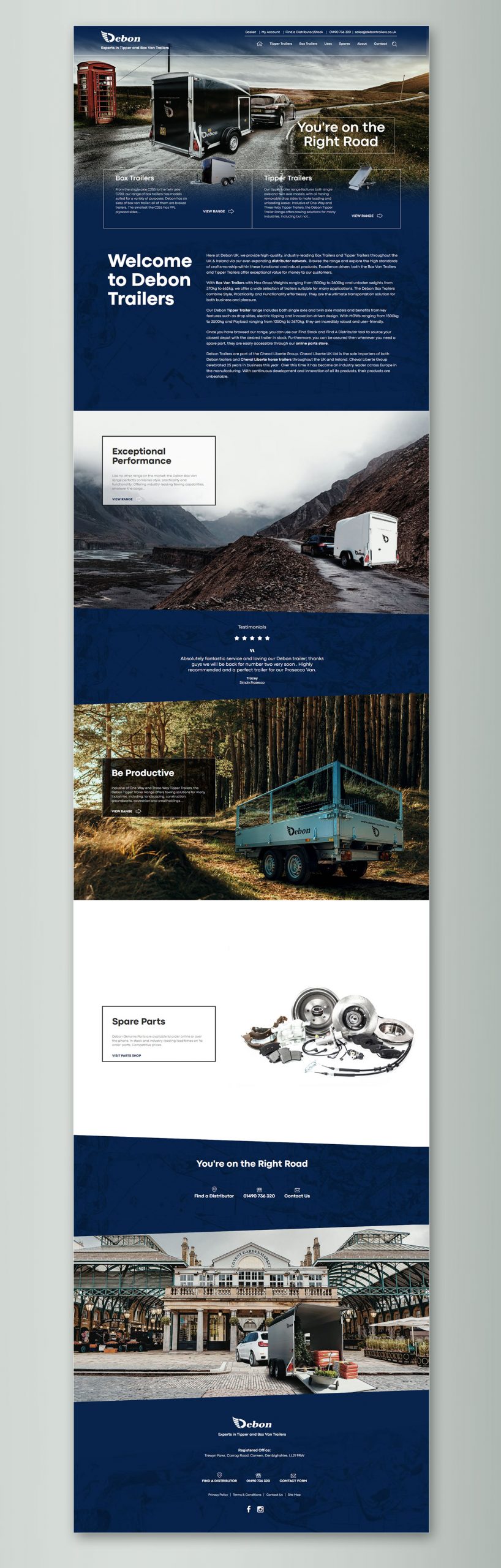The image shows a sophisticated and user-friendly website for "The Bond Trailers," specializing in tipper and box trailers. The website header includes essential navigation options such as a shopping basket, a user account section, and a "Find a Distributor" feature for locating local sellers. Additional links provide comprehensive information and access to other related websites, while a prominent home button ensures users can easily return to the main page.

The main section displays a vivid image of an SUV towing a trailer along a rocky, paved road, with a distinctive British phone booth to the left, set against a natural, serene backdrop. A prominently placed box contains the text "You're on the right road" and a comparison between box trailers and tipper trailers. It details their features and pricing options, helping users make informed decisions.

Beneath this section, a welcoming message introduces visitors to "The Bond Trailers," outlining the shop’s offerings. Further down, another captivating image showcases a trailer navigating a steep, winding mountain road with no guardrails, highlighting the exceptional performance and durability of the trailers. Testimonials and additional images provide real-world glimpses of the products in action, reinforcing the brand's reliability.

Towards the bottom of the page, users can find distributor information and contact details, ensuring easy access to customer support and sales services. The website's meticulous design and detailed content effectively convey the quality and versatility of The Bond Trailers, making it a go-to resource for trailer buyers.